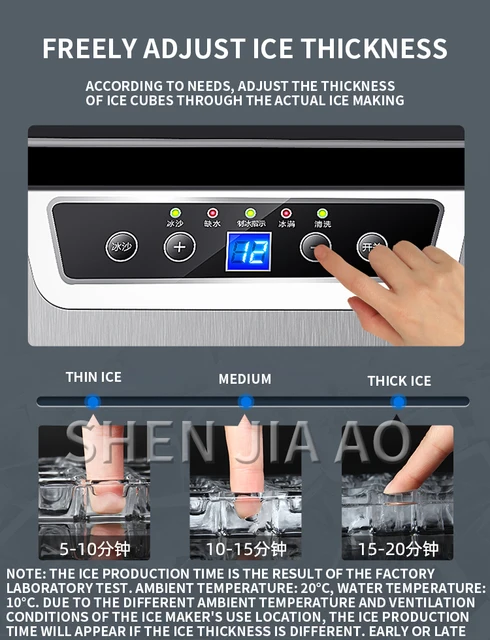This is a detailed color manual or advertisement for an advanced digital ice machine. The grey-background document prominently features a headline at the top stating, "Freely Adjust Ice Thickness." This is followed by a subheader, "According to needs, adjust the thickness of ice cubes through the actual ice making."

The centerpiece of the visual layout is a digital display on the front of the ice machine, accompanied by a hand from the right, with a single finger pressing one of the machine's four buttons. The digital readout features the number "12" prominently in its center. Below this, there's a customizable line with blue sliders that indicate three settings: "Thin Ice," "Medium Ice," and "Thick Ice." Each setting is illustrated by an image: the first showing a finger fully inserted into ice for "Thin Ice," the second showing a finger partially inserted for "Medium Ice," and the third showing a finger barely touching the ice for "Thick Ice."

Additionally, the overlay text "Shin Jia AO" is present, with further explanations of operational context beneath. There are numerical ranges (5-10, 10-15, and 15-20) next to Asian characters, and a disclosure note states, "Note the ice production time as a result of the factory laboratory test: Ambient temperature 20 degrees Celsius, Water temperature 10 degrees Celsius. Due to different ambient temperatures and ventilation conditions at the ice maker's use location, ice production time will vary if the ice thickness is different early or late."